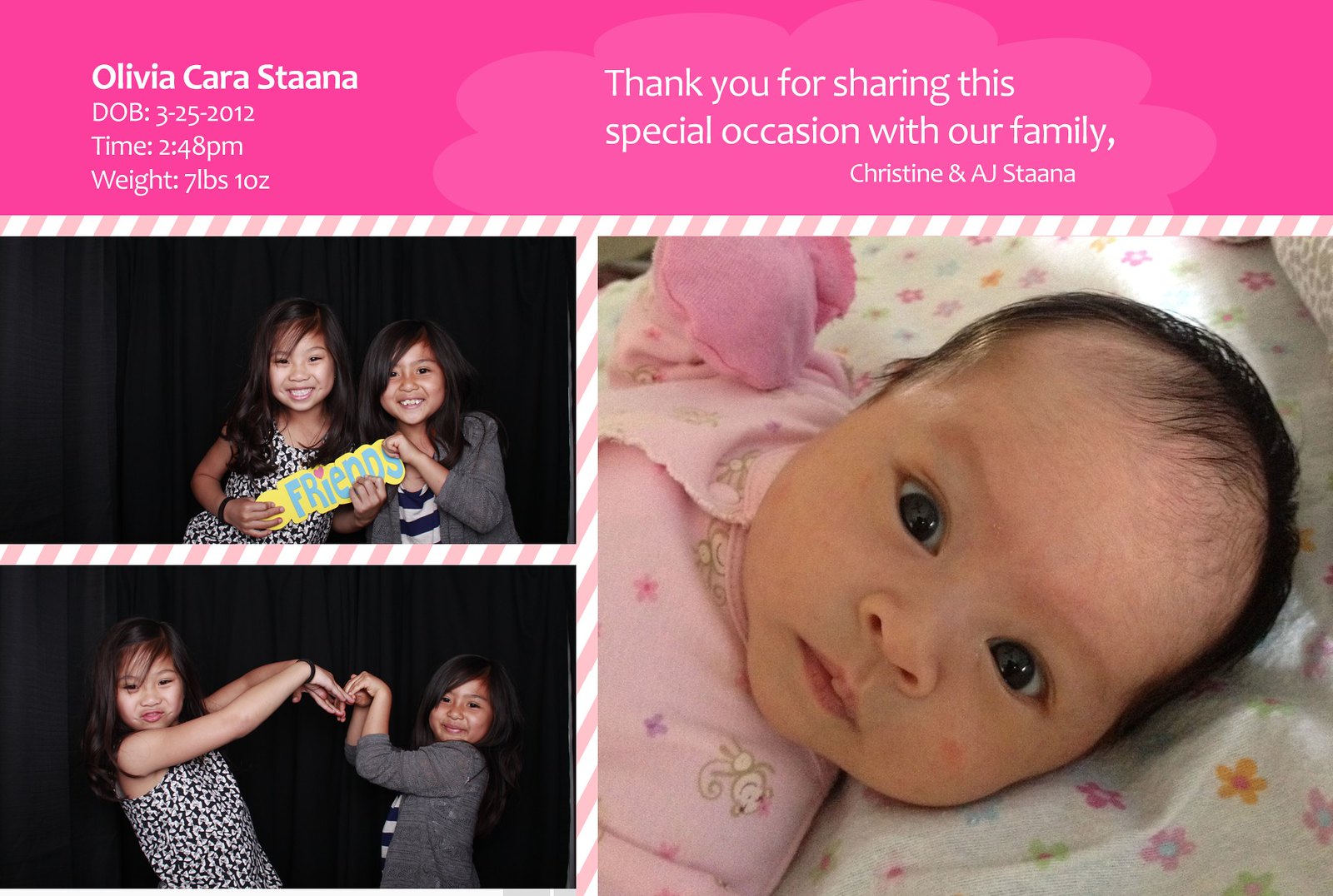This birth announcement features a full-color layout with three photographs and accompanying text set against a pink background. At the top, white text reads: "Olivia Kara Stana, date of birth 3-25-2012 at 2:48 p.m. She weighed seven pounds ten ounces." Immediately below, a message states: "Thank you for sharing this special occasion with our family. Christine and AJ Stana."

The largest photo, positioned bottom right, showcases a beautiful baby girl with dark hair and wide, expressive dark eyes. She is lying on a white sheet adorned with colorful daisy patterns in shades of pink and yellow, and she is dressed in a pink onesie.

To the left of the baby’s portrait, there are two smaller photos, one above the other. Each features two adorable young Asian girls with long dark hair. In the upper photo, the girls are holding a sign that reads "friends." The girl on the left is in a black-patterned dress, while the girl on the right wears a gray jacket over a black-and-white horizontally striped top. In the lower photo, the same two girls are seen making a playful hand gesture, touching their fingers together in a gesture akin to a high-five.